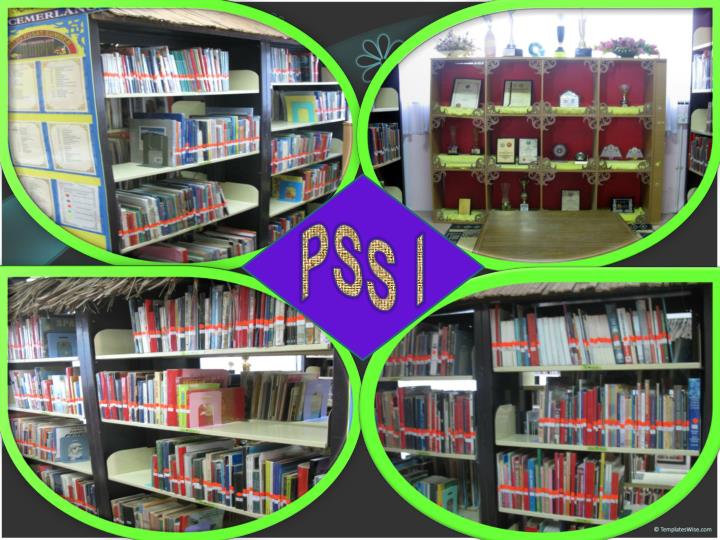The image is a digital collage composed of four distinct photographs, arranged in a grid layout with two on the top and two on the bottom, set against a black backdrop. Each photo is bordered by bright green lines, adding a striking visual separation. 

The top left photo showcases a bookshelf packed mostly with books, while the top right photo features a trophy case containing various awards and achievements. The bottom two photos also depict bookcases filled with books, reinforcing a library-like setting. Among the array of colors present in the photos are tan, black, brown, shades of red, orange, yellow, green, purple, gold, maroon, light blue, gray, and beige. In the middle of the collage, the text 'PSSI' is prominently displayed in a diamond shape, hinting at a possible presentation context.

Overall, the collage emphasizes collections of books and showcased items, presumably indoors, and appears to be a stylized portrayal possibly created through digital means.